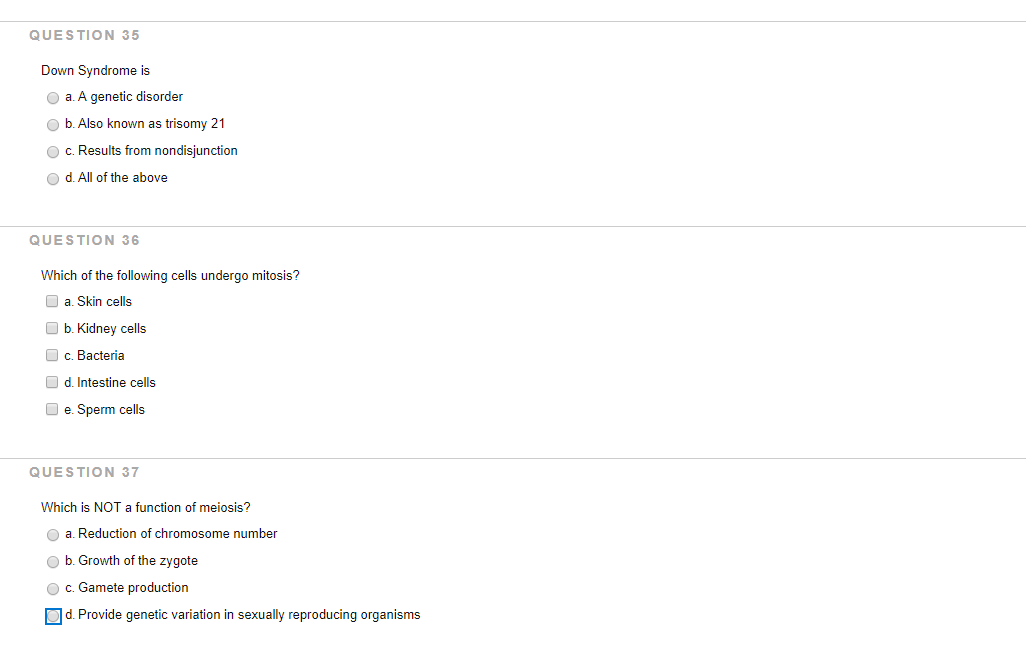The image features a white background with a fine grey line separating three multiple-choice questions. Each question is numbered, and they include "Question 35" in uppercase grey text. The questions themselves are written in black. 

Question 35 reads: "Down syndrome is" followed by four options:
A. A genetic disorder,
B. Also known as trisomy 21,
C. Results from nondisjunction, 
D. All of the above.
There is no indicated answer choice for this question.

Question 36 asks: "Which of the following cells undergo mitosis?"
A. Skin cells,
B. Kidney cells,
C. Bacteria,
D. Intestinal cells,
E. Sperm cells.
Similarly, no specific answer is selected for this question.

Question 37 inquires: "Which is NOT a function of meiosis?" with the word "NOT" capitalized for emphasis.
A. Reduction of chromosome number,
B. Growth of the zygote,
C. Gamete production,
D. Provide genetic variation in sexually reproducing organisms.
Here, option D is marked with a small blue box, indicating it has been selected.

The overall design is clean and the layout separates each question clearly, with each question containing its respective multiple-choice options listed in sequence.